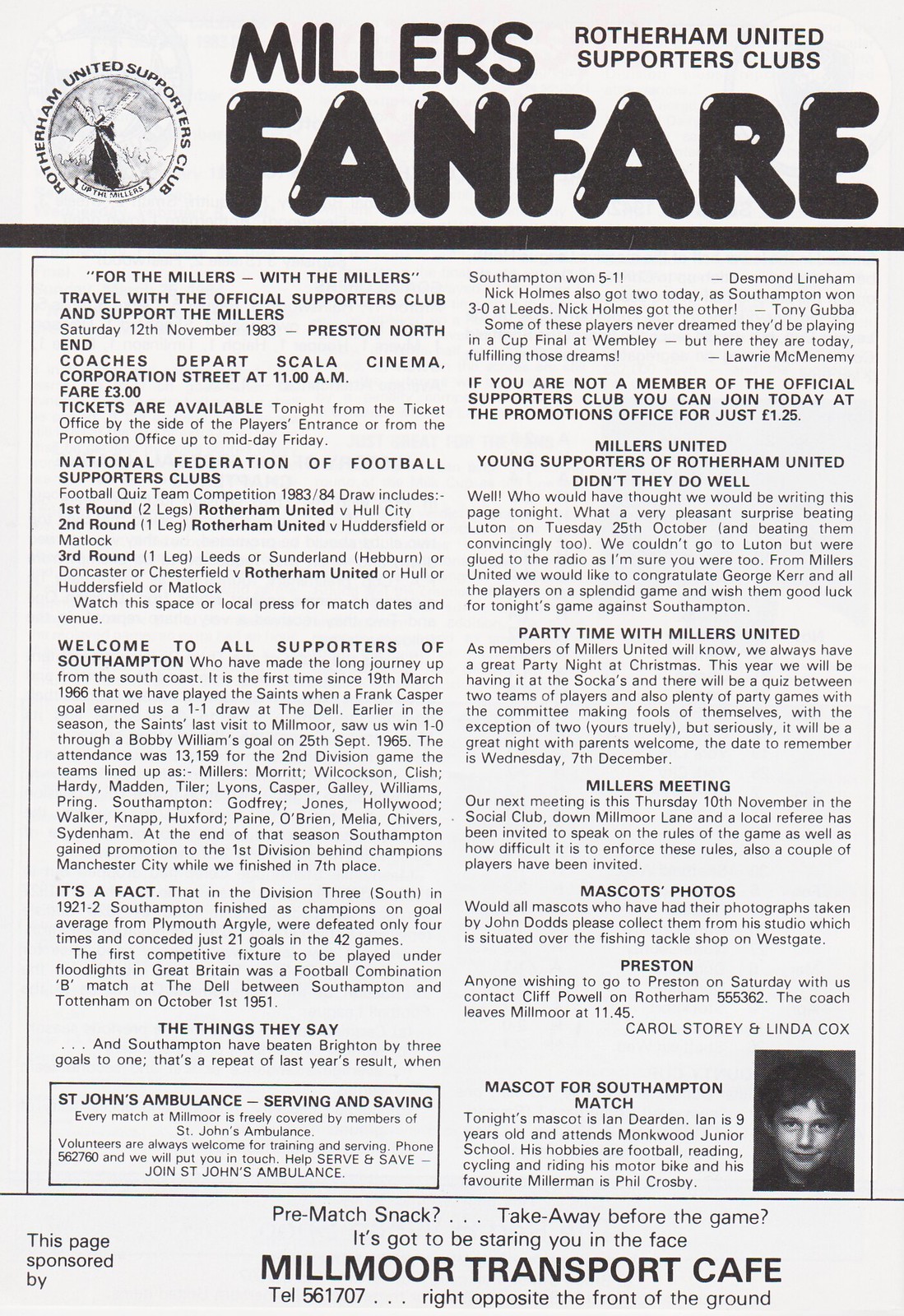The image is an advertisement or newsletter page for the Rotherham United Supporters Club, featuring detailed sections of text and graphics. In the upper left corner, a circular emblem reads "Rotherham United Supporters Club," resembling a coin. Prominently displayed in large, 3D-like black print is the title "Miller's Fanfare." Above this title is a solid black bar with the club's name repeated.

Beneath the main header, the publication features multiple sections of text. The top-most section introduces the club's purpose, stating, "For the 'Millers'," and discussing travel arrangements and support for the Millers, including cinema showings at 11 a.m. for a fare of $2.00. Tickets are mentioned as available for purchase.

Further down, the text highlights a welcome message to all supporters of Southampton and includes a reference to the National Federation of Football Supporters Club. Following this, there's a detailed breakdown of various sections such as "The Things They Say," "Millers United," and "Welcome to Young Supporters of Rotherham United," highlighting accomplishments and events.

In a right-hand column, a call to action invites non-members to join the official supporters club for $1.25 at their promotion office. Additional columns include headings like "Pretty Time with Millers United," "Millers Meeting," "Mascots Photos," and "Preston," with mentions of individuals such as Carol Story and Linda Cox, and noting a young boy as the mascot for the Southampton match.

At the bottom, a black and white picture of a young boy with black hair is featured, captioned regarding his role as the mascot. Beneath this image, another black bar leads into an advertisement for the Millmore Transport Cafe, suggesting pre-match snacks with the tagline, "Take away before the game? It's got to be staring you in the face." The cafe is described as located right opposite the front of the ground, with a telephone number provided.

The whole page has a grey background, akin to a newspaper, with the bottom left corner noting that the page is sponsored by the Millmore Transport Cafe.